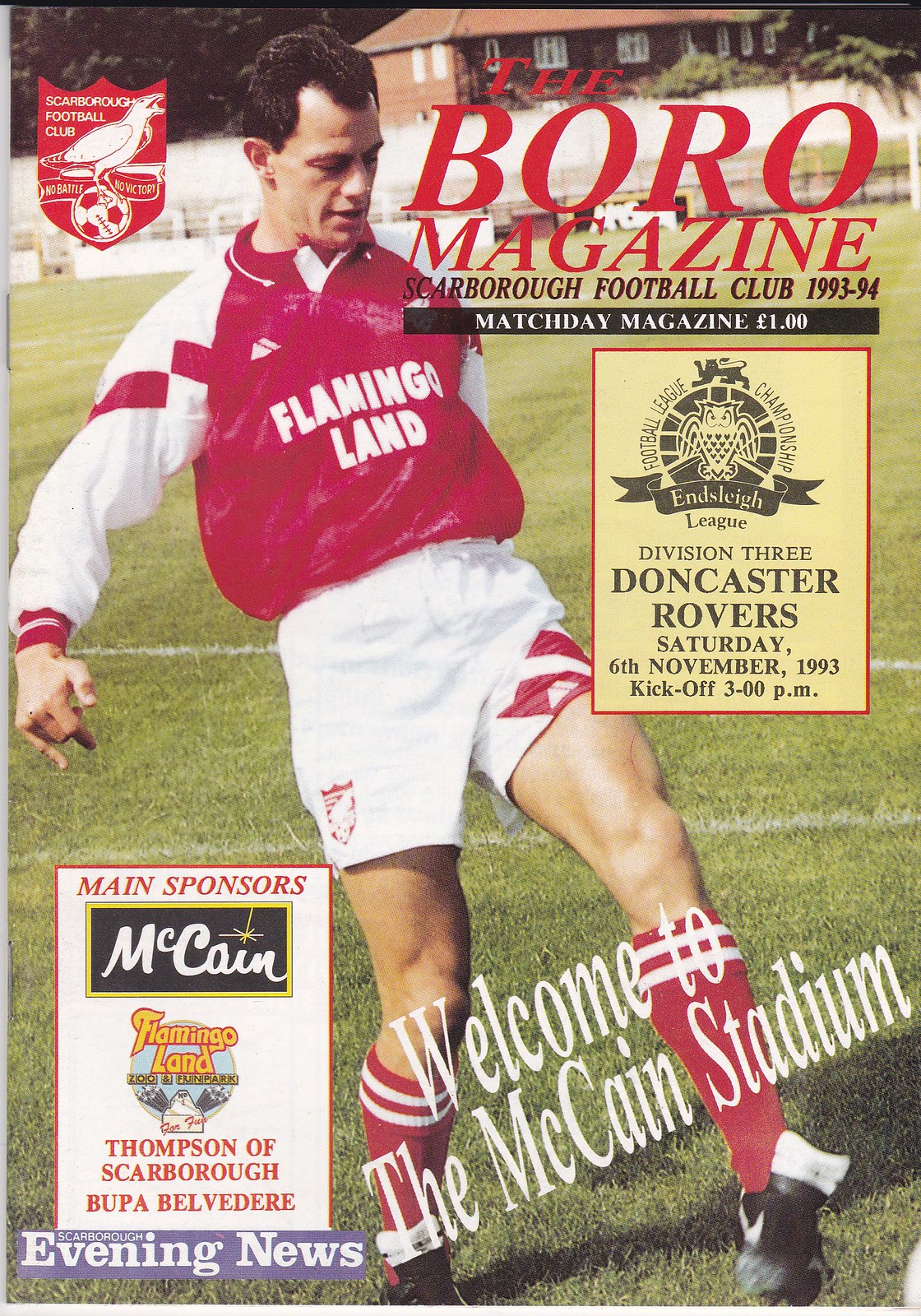The image is the front cover of "The Boro Magazine," featuring a poster advertisement for the Scarborough Football Club's 1993-94 season. Dominating the center is a footballer dressed in a red uniform shirt with white sleeves, accented by red stripes and cuffs. His white shorts are paired with red socks sporting white stripes, and he is wearing black shoes. Positioned on a green soccer field, the player appears to be mid-kick, with his left foot lifted. The player's jersey prominently displays the sponsor "Flamingo Land." 

In bold red letters at the top, the magazine title "The Boro Magazine" is inscribed, followed by "Scarborough Football Club 1993-94" beneath it in black letters. Further down, it states, "Match Day Magazine, one pound." The upper left corner features the Scarborough Football Club symbol. Moreover, the lower left corner lists the main sponsors: McCain, Flamingo Land, Thompson of Scarborough, Bupa Belvedere, and Evening News. A diagonal inscription in white letters at the bottom right corner reads, "Welcome to the McCain Stadium." Additionally, there is a rectangular section on the right side of the image that mentions an upcoming Division Three match against Doncaster Rovers, scheduled for Saturday, 6th November 1993, with a kickoff at 3 p.m. 

This detailed summary encapsulates the key visual and textual elements of the magazine cover, reflecting its vibrant sports theme and promotional content.